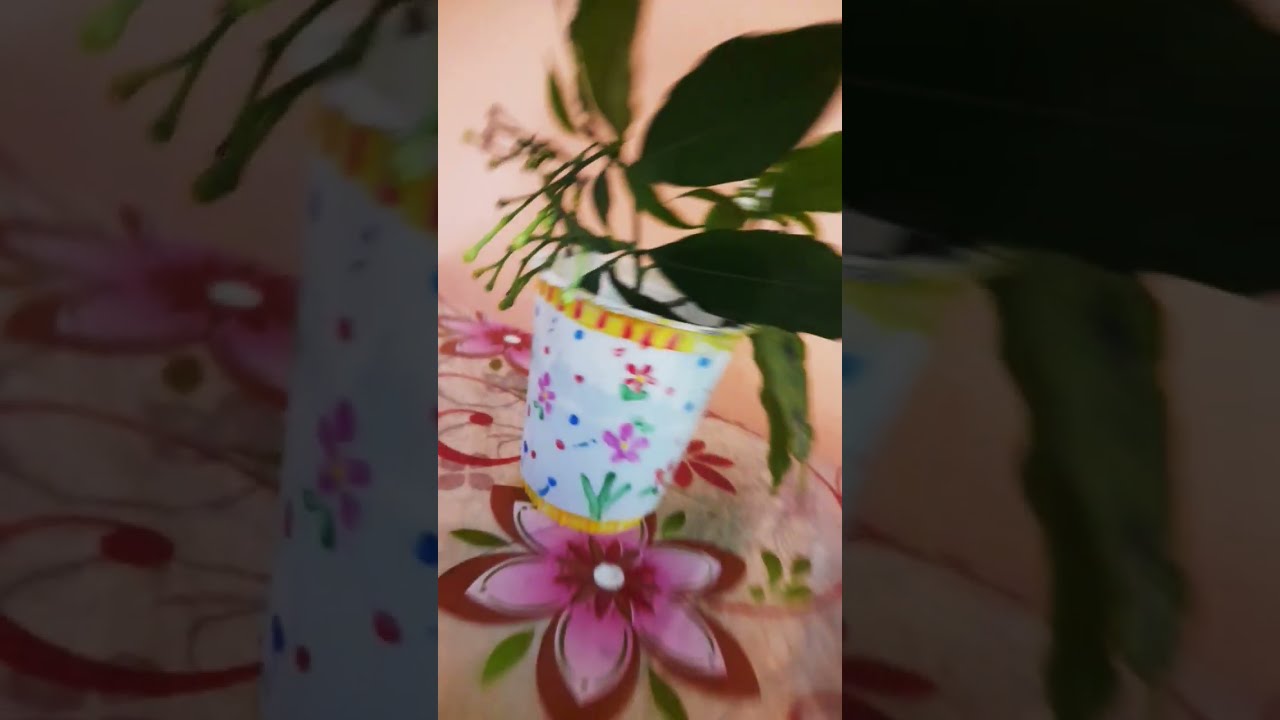The image features a vertically cropped photograph, likely taken on a smartphone, showcasing a healthy potted plant placed on a glass table with intricate floral designs. The pot, centered in the image, is predominantly white with multiple decorative elements, including pink and red petal flowers with yellow centers, green stems, blue dots, and a yellow band with red vertical stripes at both the top and bottom. The plant itself, boasting dark green leaves, appears lush and vibrant. The glass table below it is adorned with a flower print showing large pink blossoms with red outlines and green accents. In the blurred background, there is a soft pink or peach wall. The photo has a light center with darker, more zoomed-in borders on the left and right, adding depth to the composition.